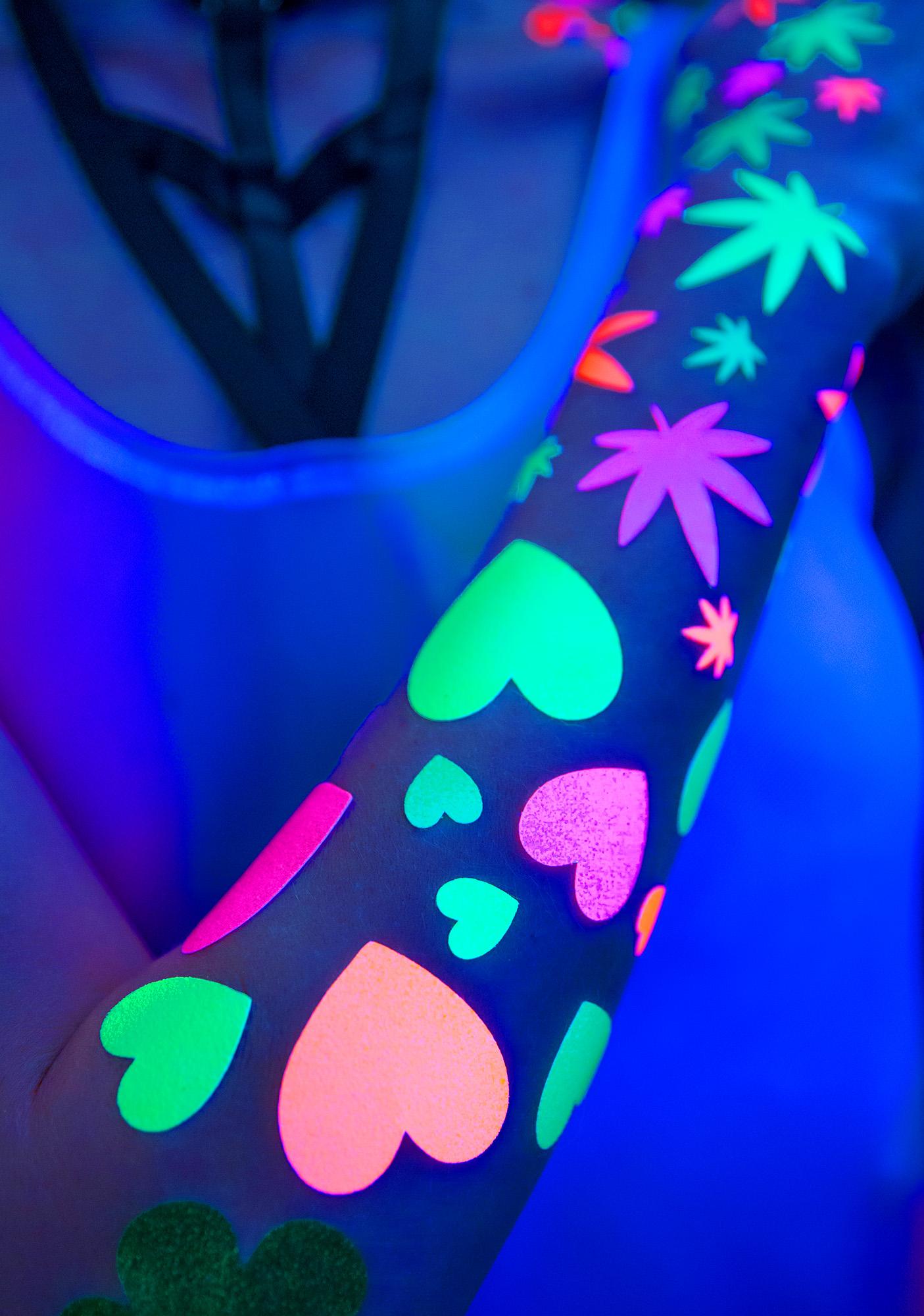In a dimly lit room with a blue-black light casting a glow, the photograph focuses on a young woman's right arm, which is prominently displayed and nearly fills the frame. Her arm is adorned with a variety of vividly colored stickers, including hearts in shades of peach, green, pink, and purple, as well as assorted leaves—some of which resemble marijuana leaves—in hues of green, purple, and orange. These stickers cover her entire forearm and hand, from right above her elbow to just below her knuckles. She is wearing a white semi-transparent shirt over a black garment, which complements a thick black collar around her neck. The rest of her body is partially visible in the blurred background, emphasizing the detailed and colorful decoration on her arm.